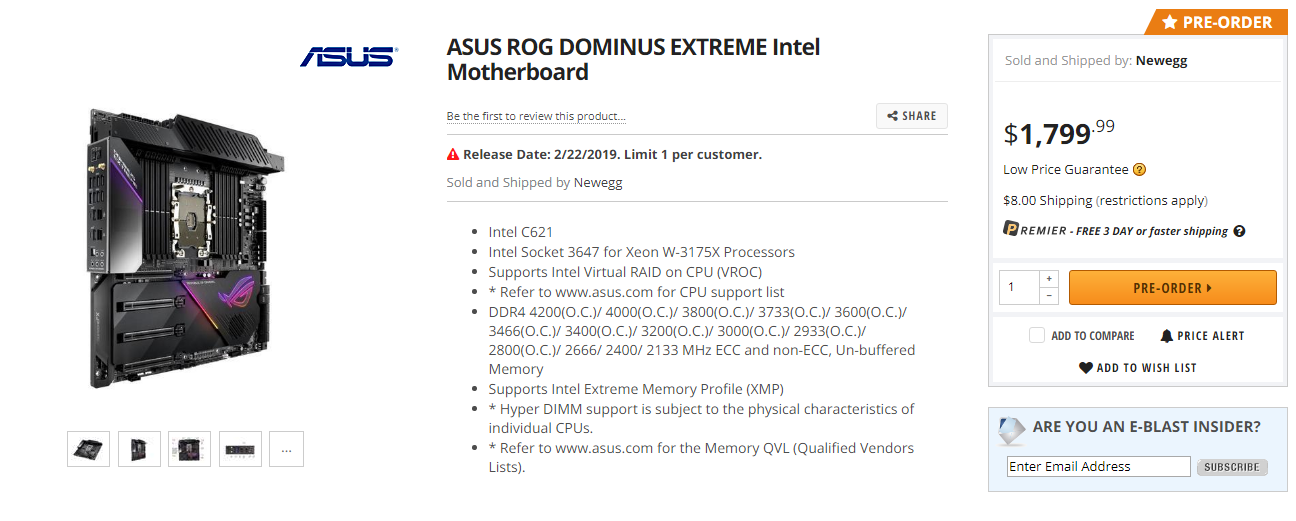Screenshot capturing the detailed page of an Asus ROG Dominus Extreme Intel Motherboard on Newegg. The main image prominently displays a side view of the high-end motherboard, accompanied by several smaller thumbnails underneath that allow users to explore different angles and aspects of the board. The page features a pre-order button, indicating the motherboard is available for pre-order at a price of $1,799.99. The mention of "E-Blast Insider" suggests a promotional newsletter from Newegg. The motherboard specification implies compatibility with Intel processors, likely targeting the i9 series, as suggested by the detailed description and numerical specifications. The product is explicitly noted to be sold and shipped by Newegg.